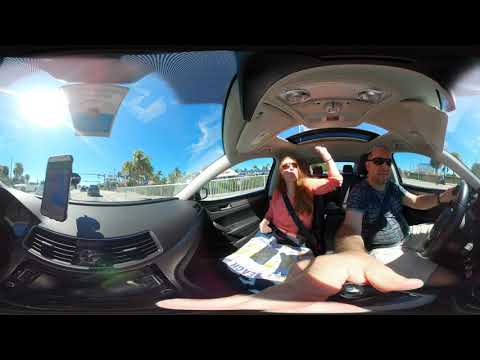In this panoramic 360-degree image taken from inside a car, you see a detailed view of the vehicle's interior and its occupants. On the right side, a woman with long brown hair, wearing sunglasses and a light pink long-sleeved top, is sitting in the passenger seat. She has her seatbelt fastened and appears to be engaging with a map. Her hair drapes over her shoulder. Her left hand is reaching towards the sunroof, which is partially open, allowing sunlight to filter into the car.

Next to her, the driver, an older man with a slightly protruding belly, is wearing a blue shirt, khaki shorts, and sunglasses. His left hand is firmly on the round black steering wheel, while his right hand, wearing a black watch, holds the camera that took the panoramic image. The dashboard in front of them shows AC vents and a cellphone mounted on a holder. There's also a tag hanging from the rearview mirror. Outside the windshield, the clear blue sky is dotted with clouds, and you can see trees and other cars on the road. The sun sits prominently near the top of the windshield, casting a bright light throughout the car. The back seats and more of the blue sky are visible through the rear windows, completing the scenic and immersive view from within the car.